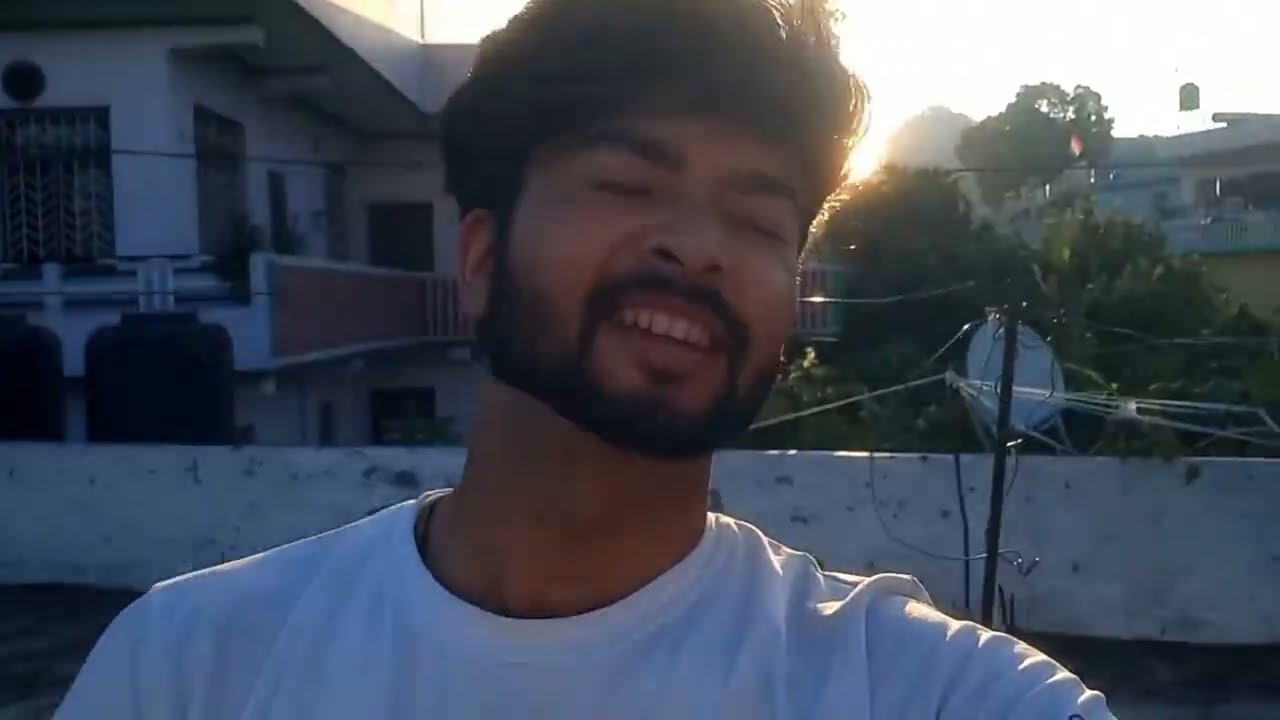The photograph is a slightly blurry, close-up image of a young man with brown skin and dark features, taken outdoors on a sunny day. He's smiling with his mouth open, showing his upper teeth, and his eyes are closed. He has a full, black bushy beard and mustache, and his thick, dark hair extends out of the frame at the top. He's wearing a white crew-neck t-shirt and appears to be taking the photo himself, with his left shoulder slightly extended forward. His head is tilted back and to the right, catching some of the bright sunlight that makes the sky appear hazy and white. In the background, there are white buildings to the left and right, including a two-story building with an orange side and a balcony. Behind the man, there's a white stone wall with trees and power lines visible above it, suggesting he might be standing on a rooftop in a residential area, possibly in Asia. A satellite dish can also be seen on the right-hand side behind him. The bright sun near the horizon adds a warm glow to the scene.